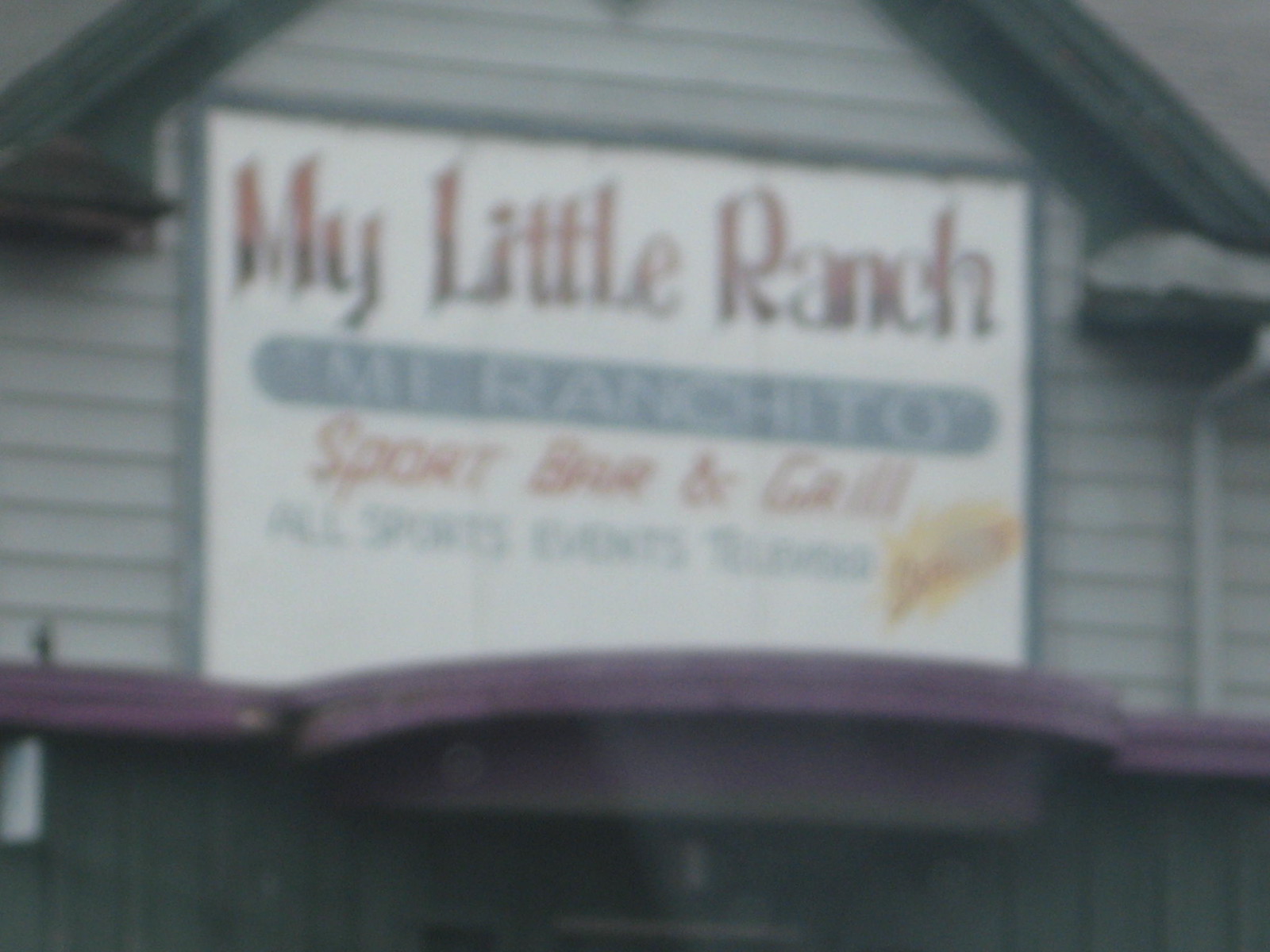This photograph is a close-up, cropped image of the front of a building, though it is somewhat blurry. The focus of the photograph is on a large advertisement sign for "My Little Ranch, Sports Bar and Grill." The sign itself is white with bold red text. There is additional text on the sign, but due to the blurriness of the image, it is difficult to decipher. A yellow logo is visible in the bottom right corner of the sign. The advertisement is mounted on a grey building constructed from wooden planks. This descriptively captures the essence of the scene despite the image's lack of clarity.